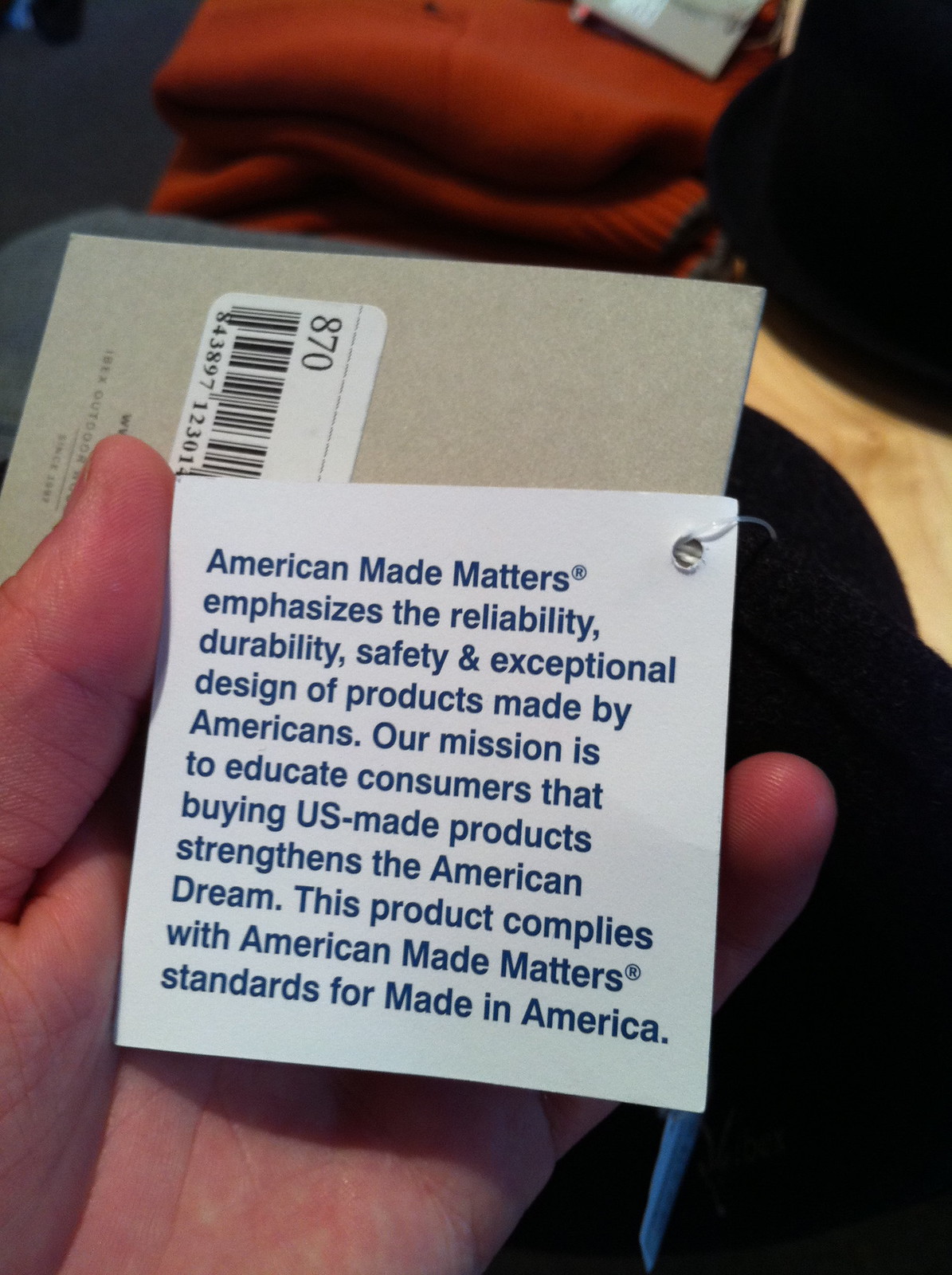A detailed close-up image showcases a person with fair skin holding multiple tags in their hand. The prominent tag is white and square-shaped, bearing the text: "American-Made Matters emphasizes the reliability, durability, safety, and exceptional design of products made by Americans. Our mission is to educate consumers that buying U.S.-made products strengthens the American Dream. This product complies with American-Made Matters standards for Made in America." In the background, red fabric garments are neatly folded and stacked, accompanied by a light-colored wooden hanger, adding context and depth to the scene.